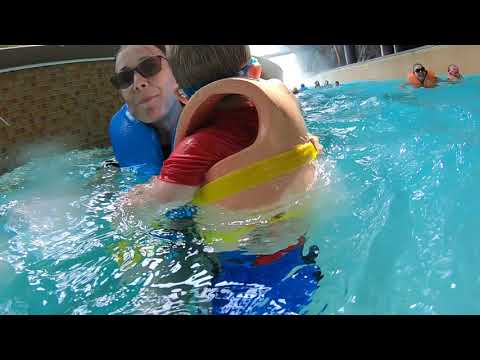In this pixelated and blurry still from a video, a lively water park scene is captured. The image focuses on a woman wearing sunglasses and a blue life vest as she holds a small boy, estimated to be around three to four years old, who is clad in an orange life vest with yellow straps and blue swim trunks. Water droplets on the camera lens add a touch of realism to the clear, bright blue water that characterizes this lazy river ride, surrounded by concrete sides in a peach color and bordered by tiles in brown, tan, and white hues. Behind this pair, another woman in an orange life vest is visible, also guiding a boy of similar age in a yellow life vest. Further along the river, approximately five more individuals can be seen enjoying the ride, emphasizing the busy and joyful atmosphere of the water park.